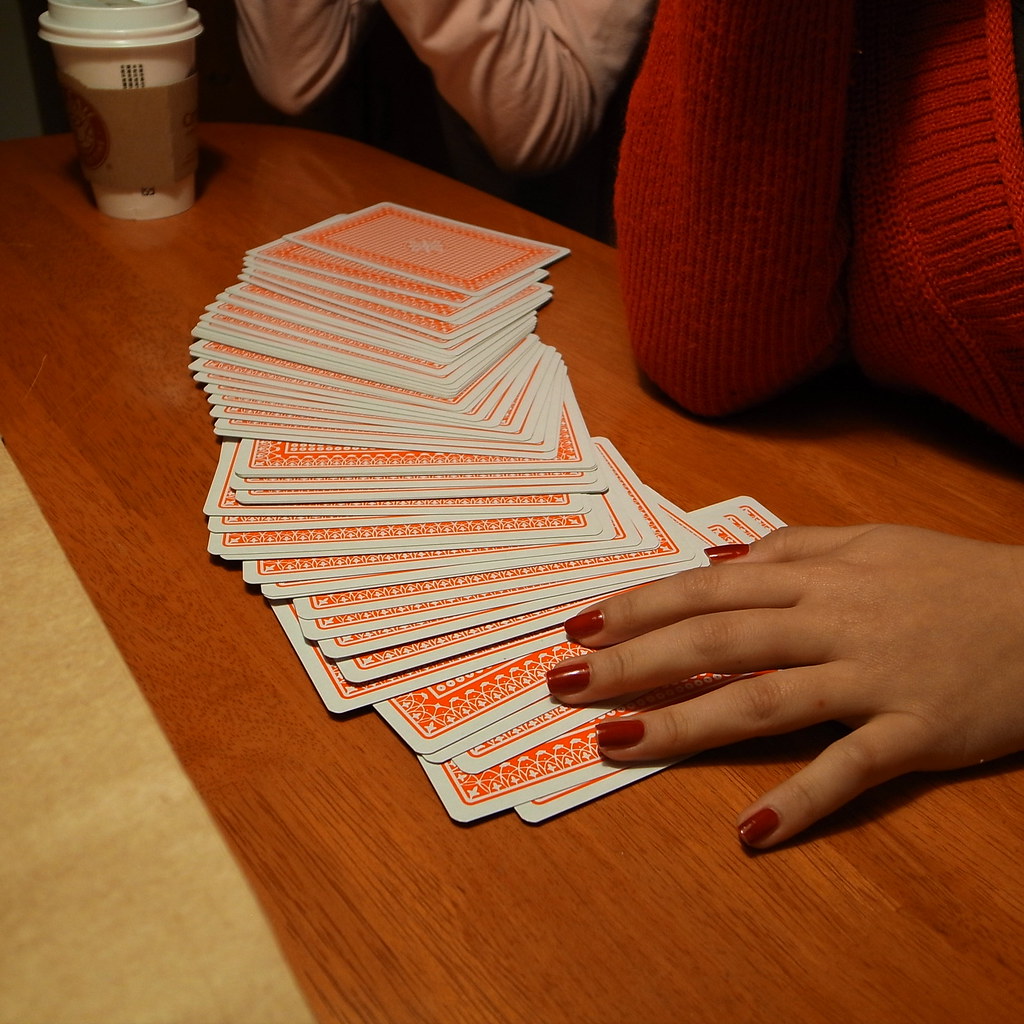In this photograph, there's a slightly visible countertop above a table. A woman's hand, adorned with red nail polish, rests on a spread-out deck of cards. Her elbow is placed on the table directly in front of the cards. She wears a red sweater, which is cast in a gentle shadow. Beside the cards, a cup of coffee is placed. Another woman, visible only from her elbows wearing a long-sleeved pink shirt, appears to be engaged with the scene. The image captures a moment of stillness, with the first woman's hand poised as if she is about to select a card, and the second woman's posture hinting at anticipation.